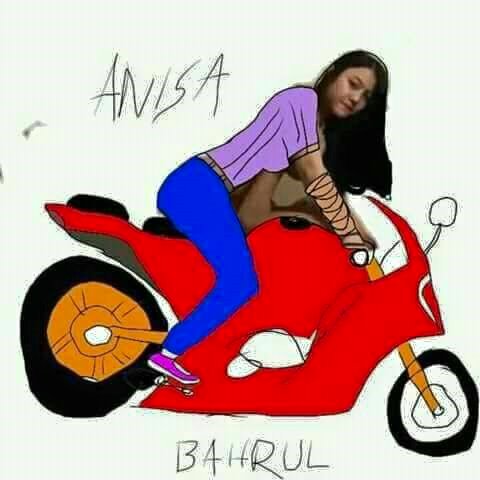The image is a composite of a child's hand-drawn motorcycle and a real-life photo of a woman. The motorcycle, rendered in red with an asymmetrical design, features a large back wheel with an orange rim and a smaller front wheel with a white rim. It has two seats and includes details like a forward-leaning windshield and a side mirror. The child's handwriting labels the image with "Anissa" at the top and "B-A-H-R-U-L" at the bottom. 

The main subject is a woman on the motorcycle, depicted with a combination of hand-drawn elements and a cut-and-paste photograph. She is wearing pink shoes, blue jeans, and a purplish top. Her head and arms are taken from an actual photo, resulting in a somewhat crude and poorly photoshopped appearance. She has long dark hair that reaches down to the windshield, and her head angle suggests that the original photo was possibly from an adult film, as inferred from the visible supporting arms beneath her. The background is an off-white color, adding to the makeshift and child-like aesthetic of the entire composition.